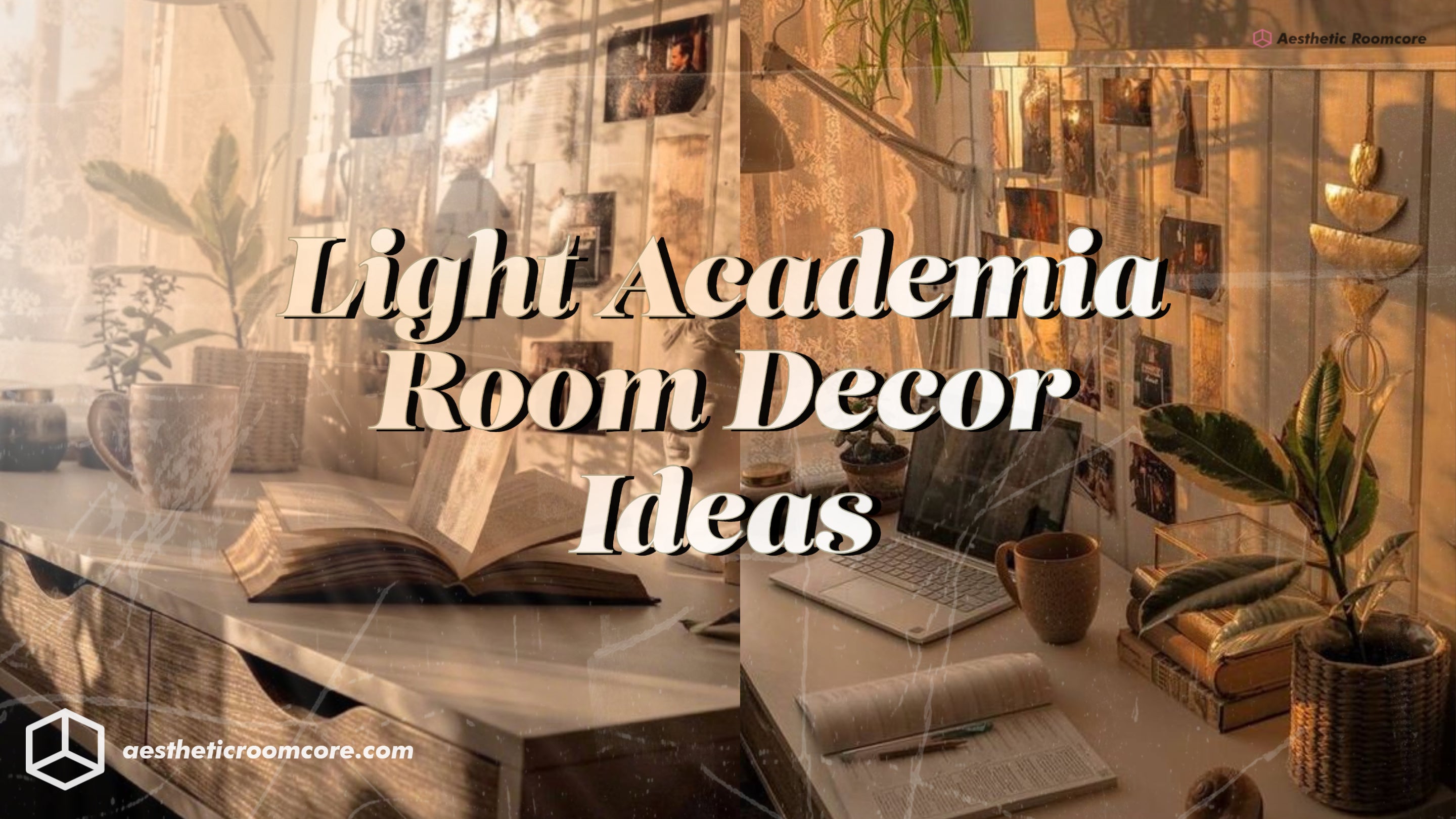The image depicts a dimly lit room with a warm brownish tone, suggestive of the Light Academia aesthetic. Dominating the left side of the room is a white-topped desk featuring an open hard-bound book and surrounded by lush greenery. Behind the desk, a bulletin-like board displays several indistinct pictures and decor items, hinting at a purposeful but subtle organization. The right side of the room is centered around another desk with a wooden finish, adorned with an open laptop, a coffee mug, and a partially open soft-bound book weighed down by some pens. Additionally, three hard-bound books are neatly stacked nearby. The room is embellished with hanging decor, including a distinct piece comprised of four horizontally aligned segments of increasing size from top to bottom. Adding to the room's charm is a multitude of plants and numerous photographs lining the wooden wall, contributing to a tasteful, albeit slightly cluttered, ambiance. A stylistic overlay gives the whole image a crackled texture, enhancing its vintage aesthetic. Overlaying the scene are the words “Light Academia Room Decor Ideas” in white font, and the bottom left corner bears the logo “AestheticRoomCore.com.” The overall image appears to be an advertisement, akin to an Ikea catalog, offering decor inspiration with an emphasis on a cozy, intellectual atmosphere.